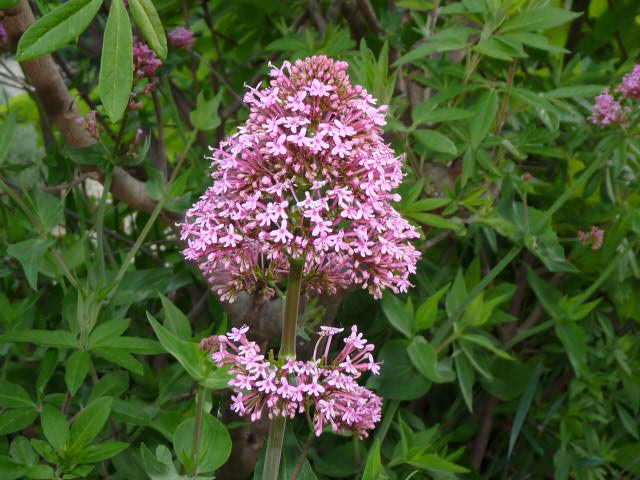In this daytime garden scene, a flowering plant with green leaves and pink blossoms captures the eye. The plant features multiple stems, with one particularly strong green stalk supporting clusters of vibrant pink flowers and budding blooms, suggesting a thriving lilac or possibly goldenrod plant. Surrounding this primary stalk, other green leaves and smaller stems contribute to the lush foliage. In the background, additional similar flowers and a few bushes can be seen, adding to the garden's verdant tapestry. A noticeable one-inch-thick branch rises from behind the flowering plant, possibly part of a small tree, which adds complexity to the composition.